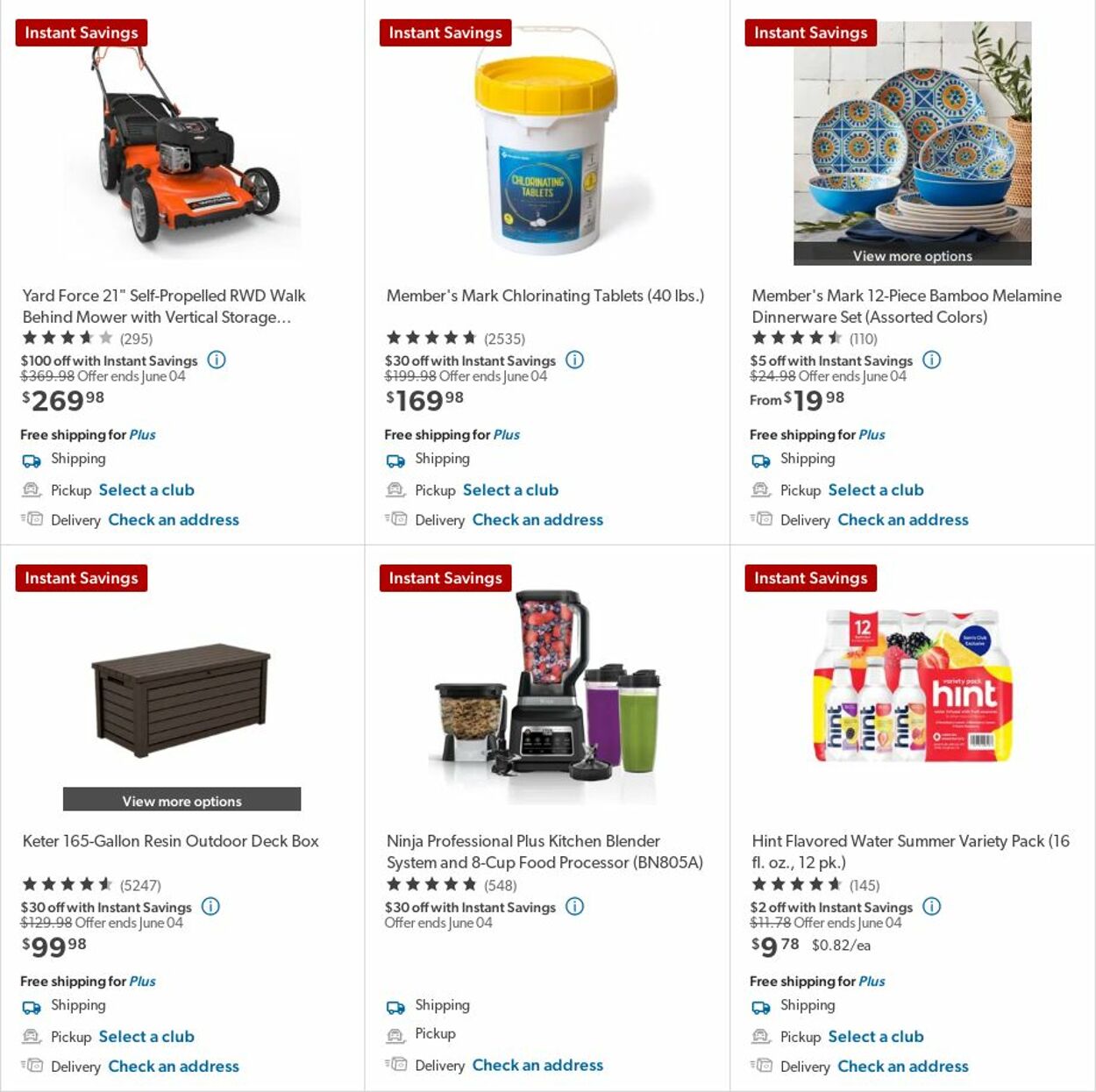This image appears to be a promotional snapshot from a shopping website, likely resembling a layout from Costco or Sam's Club, although the exact website is not specified. The page features enticing "Instant Savings" offers prominently showcased above each product image. The products displayed include six diverse items: a lawnmower, chlorine tablets, a colorful 12-piece bamboo dinnerware set, an outdoor deck box, the Ninja brand professional kitchen blender system equipped with an 8-cup food processor, and a Hint flavored summer water variety pack. Beneath each item, pricing details are clearly visible. The platform offers flexibility in shipping options, allowing users to choose either pickup or delivery services. Users can select their preferred club location, which reinforces the likelihood of the website being Sam's Club. The overall design suggests a user-friendly interface, emphasizing convenience and savings for shoppers.